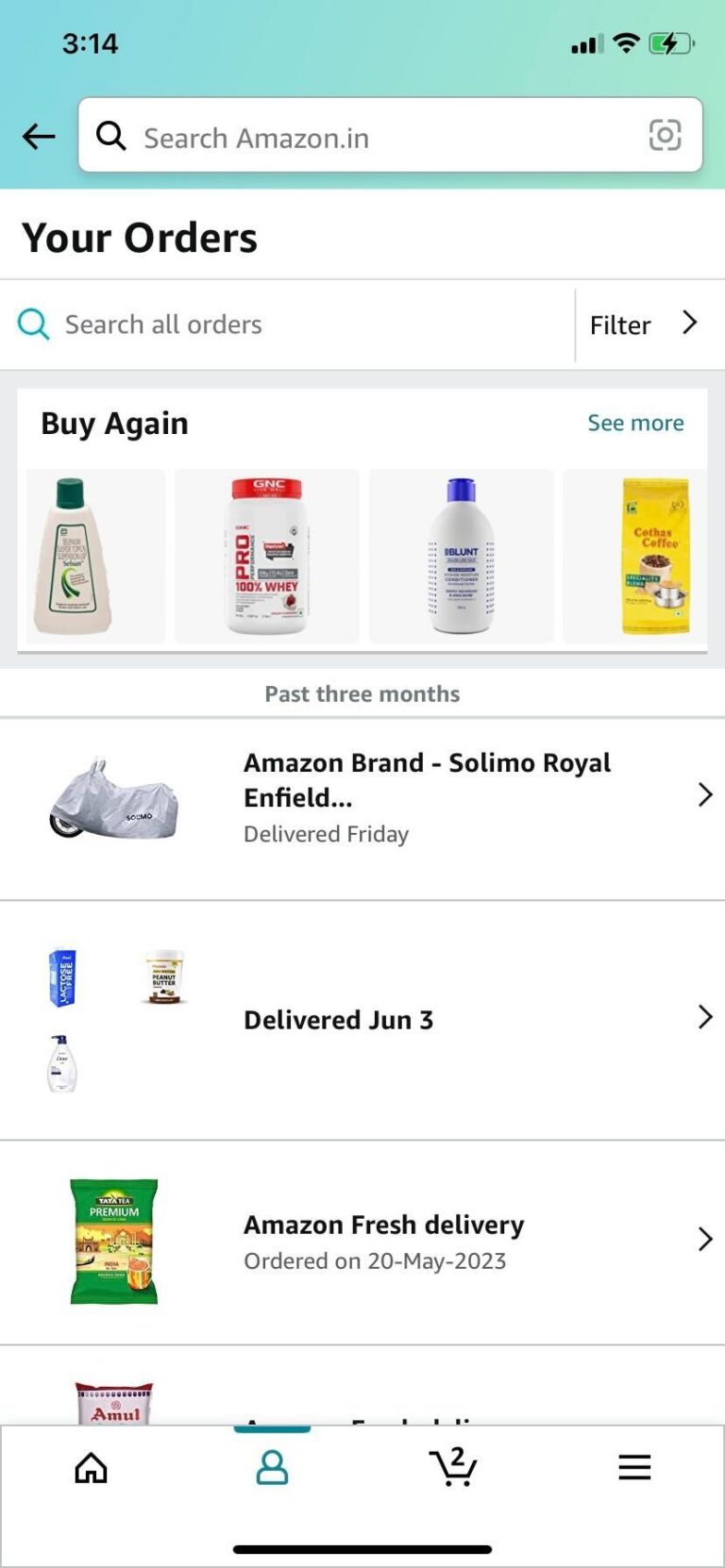This image is a detailed screenshot of an Amazon.in app displayed on a cell phone screen. The time shown is 3:14, and the status icons for cell phone reception, Wi-Fi, and battery are present at the top. Immediately below, the Amazon search bar is visible, labeled "Search Amazon.in."

Beneath the search bar, the "Your Orders" section is displayed, accompanied by another search bar labeled "Search All Orders" and a filter button. Following this, the "Buy Again" section appears, showcasing four reordered items. Among them, three items are bottles, and the fourth item appears to be a bag of coffee.

The list is organized under the "Past Three Months" heading. The first item listed is an Amazon-brand product labeled as Salamo Royal Enfield, which was delivered on a Friday. Just below that entry are three icons representing items delivered on June 3rd. Further down, there is an entry for an "Amazon Fresh Delivery," ordered on May 20th, 2023.